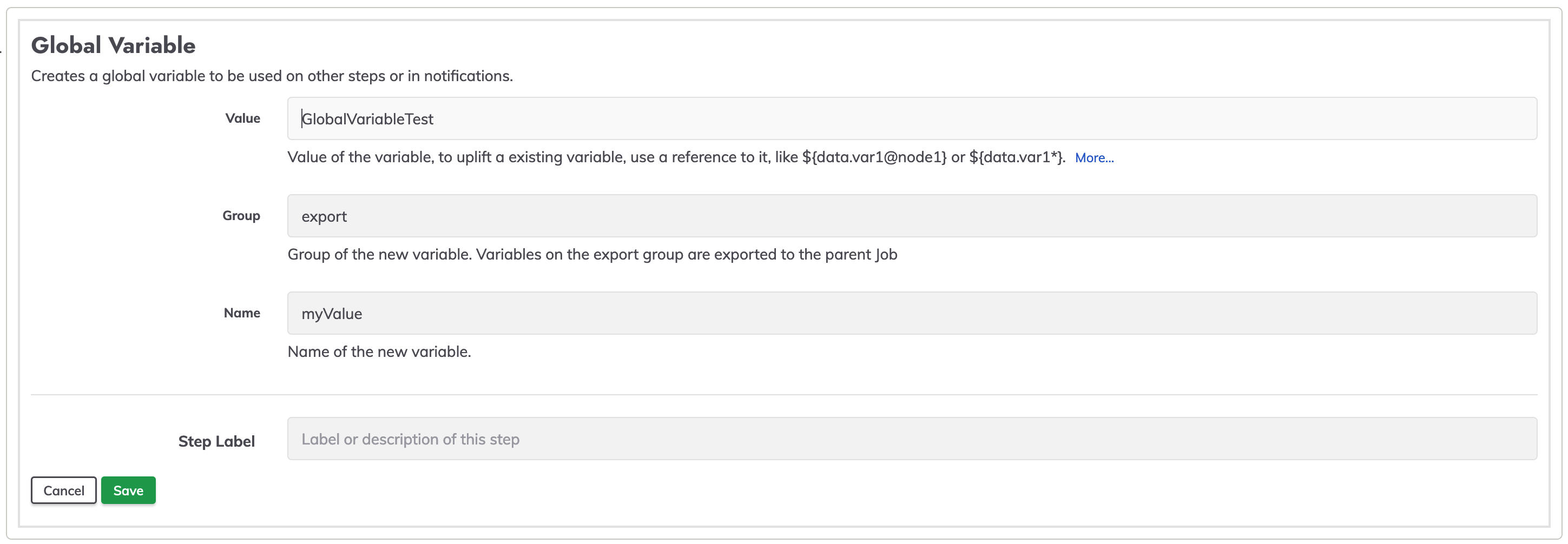This is a screenshot from a website featuring a form designed to create a global variable. The form is positioned against a white background and enclosed within a rectangle with a light gray border. At the top left of the rectangle, "Global Variable" is prominently displayed in bold black letters. 

Beneath this title, a description reads: "Creates a global variable to be used in other steps or notifications." Following this, there is a labeled section with the word "Value" accompanied by a space to input text, currently containing the placeholder "global valuable test."

Below this input field, additional instructions specify: "Value of the variable. To refer to the value of an existing variable, use a reference such as data.mail@domain.com."

Further down, there is a "Group" field with an explanation: "Export group of the new variable. Variables in the export group are exposed to the parent job." This is followed by a "Name" field with a blank space for naming the variable.

At the bottom of the form, there is a "Step Label" field with an area for input. On the lower-left corner of the form, there is a "Cancel" button, and next to it, a green "Save" button.